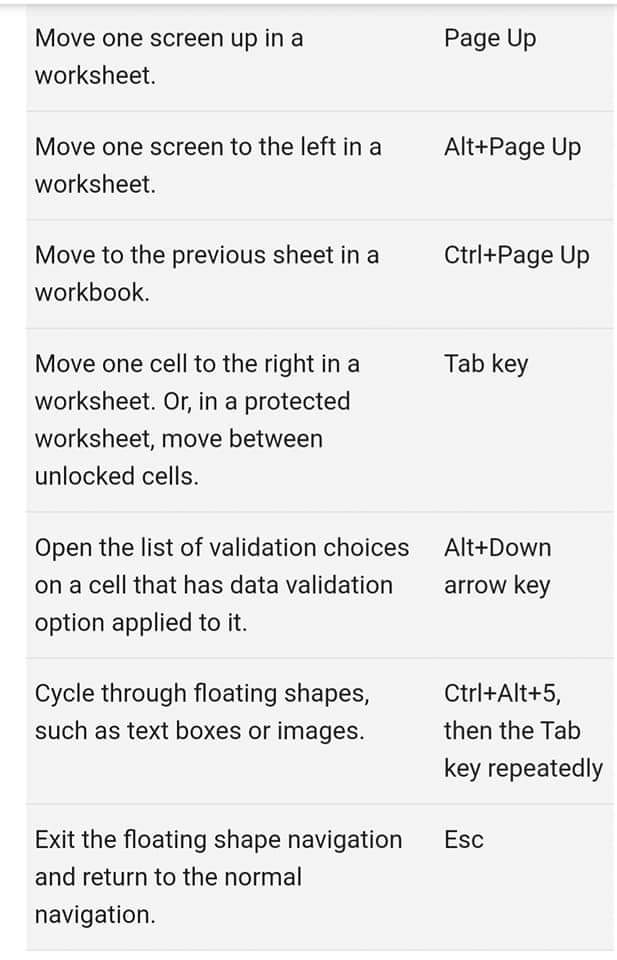This image displays a screenshot against a light gray background, featuring a list of keyboard shortcuts for navigating within an Excel worksheet. The text is entirely in black and starts with the heading "Move one screen up in a worksheet" followed by the corresponding shortcut "Page Up" on the right. 

Below that, it specifies "Move one screen to the left in a worksheet" and the shortcut "Alt + Page Up" to its right. Next, the instructions "Move to the previous sheet in a workbook" are provided, with the shortcut "Ctrl + Page Up" beside it.

Further down, you can see "Move one cell to the right in a worksheet, or in a protected worksheet, move between unlocked cells" paired with the "Tab" key. The next line says, "Open the list of validation choices on a cell that has data validation option applied to it" with the shortcut "Alt + Down Arrow Key."

Lastly, the screenshot includes "Cycle through floating shapes, such as text boxes or images" with the shortcut "Ctrl + Alt + 5." It specifies that repeatedly pressing the "Tab" key continues the cycle. At the very bottom, the instruction is "Exit the floating shape navigation and return to the normal navigation," followed by the "Escape" key.